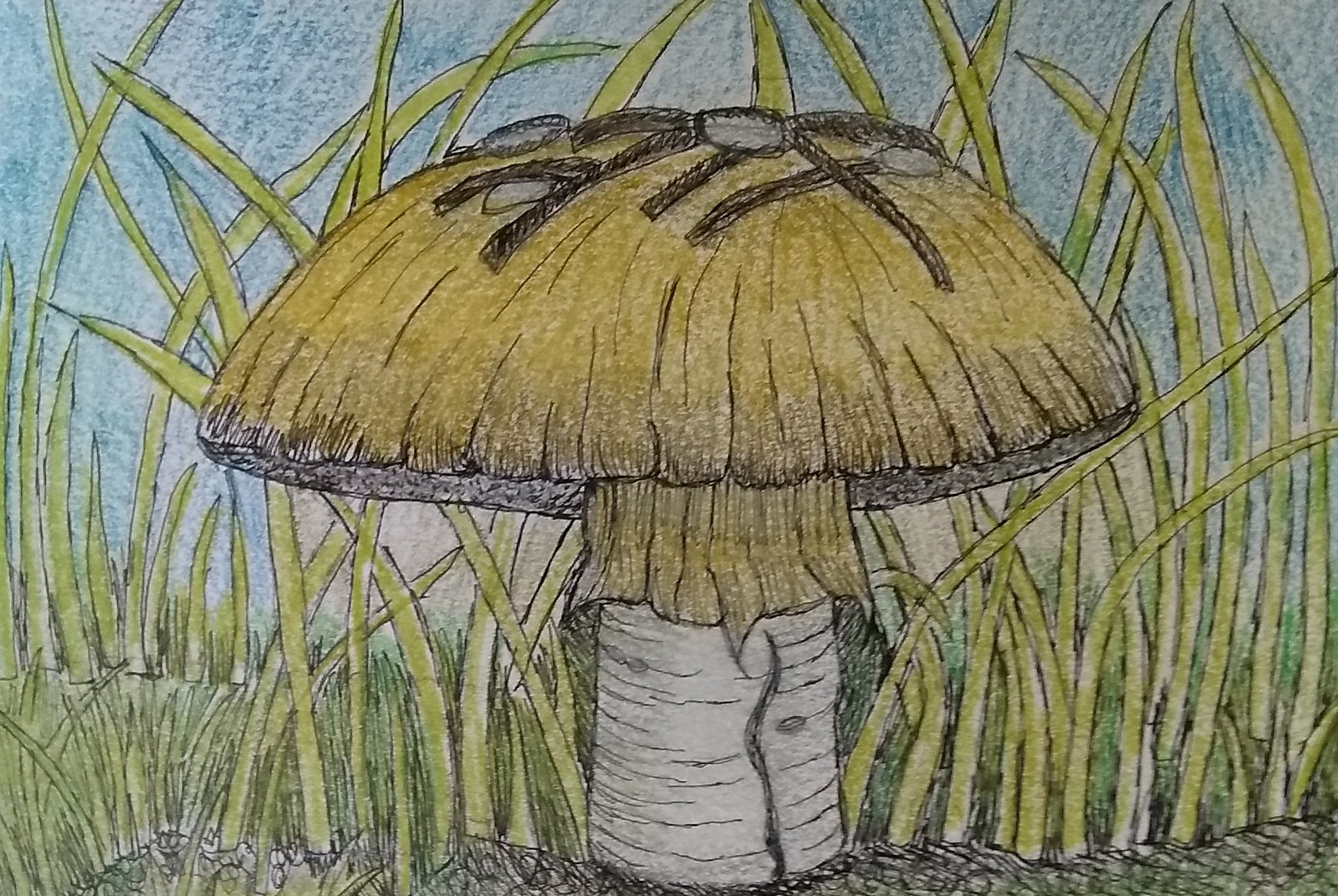Title: "Spider Resting on Mushroom in Grass Field"

Caption: 
In this rectangular drawing, the long side extends from left to right, capturing a serene scene set in a grass field. At the center of the composition stands a mushroom characterized by a light gray stem, which extends from the base up towards the midpoint of the image before transitioning into the cap. The mushroom cap, shaped like a semi-circle or oval, boasts a muted greenish-brown hue adorned with vertical lines that add texture and detail. Perched atop the mushroom cap is an intricately drawn black spider, depicted with slender lines and small circles representing its legs and body, as if taking a momentary rest. A single, curvilinear mark winds through the gray stem, adding further interest to the mushroom's structure. Surrounding the mushroom are blades of grass varying in height, painted in shades of green that bring the field to life. The backdrop reveals a peaceful blue sky, completing the idyllic and natural setting of this detailed artwork.